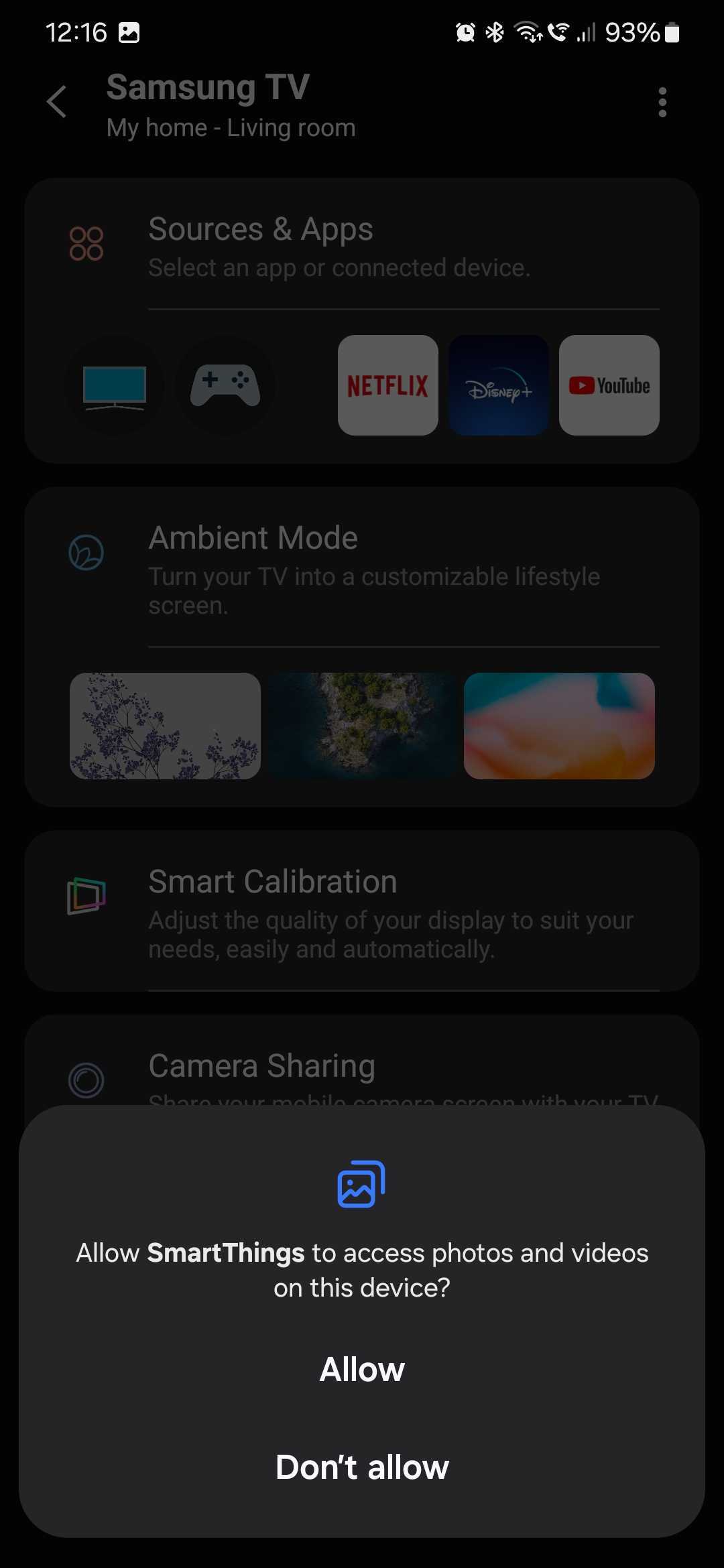The image is a screenshot from a smartphone, displaying a single long column against a black background. 

At the very bottom, there is a rounded rectangle with a slightly lighter shade of black, resembling a pop-up message. This pop-up has a blue icon featuring a mountain and a small sun. The text in bold reads: "Allow SmartThings to access photos and videos on this device," followed by two options: "Allow" and "Don't Allow."

The upper part of the blurred screen shows several elements clearly identifiable. In the upper left corner, the time is displayed as "12:16" accompanied by the SmartThings icon. The upper right corner contains standard phone status icons, including a battery icon indicating a 93% charge.

In successive rows, the content is as follows:
1. "Samsung TV, My Home, Living Room."
2. "Sources and Apps. Select an app or connected device."
3. Icons and names for various services: a monitor icon, a game, "Netflix," "Disney," and "YouTube."
4. "Ambient Mode. Turn your TV into a customizable lifestyle screen," alongside three ambient images.
5. "Smart Calibration. Adjust the quality of your display to suit your needs easily and automatically."
6. "Camera Sharing."

At the bottom, partially obscuring the content above, is the SmartThings pop-up message described previously.